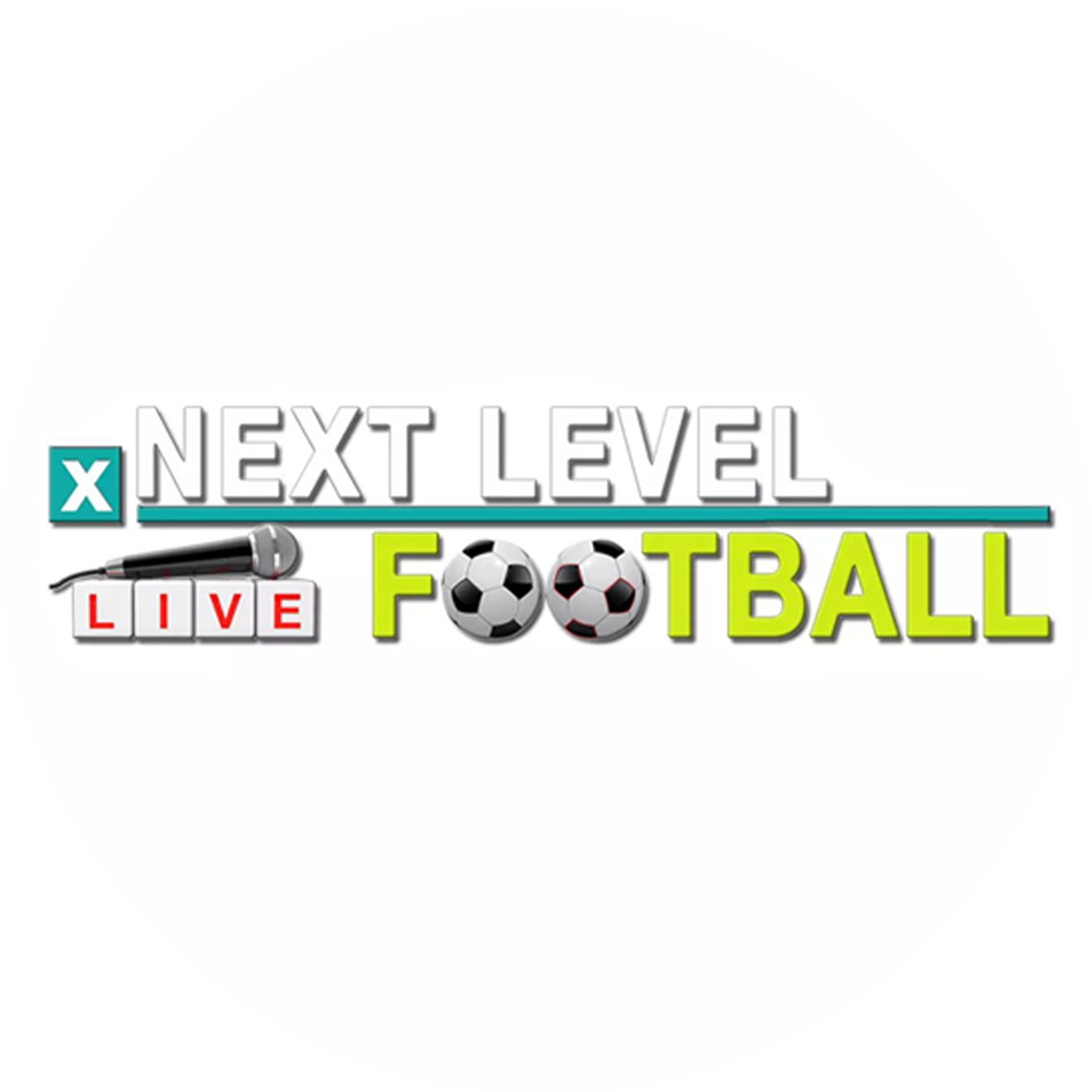The image is an infographic banner with a focus on a sports-related talk show about football, presented on a pure white background. The design is horizontally oriented and features a few key graphic elements. 

At the top, in large uppercase letters with a gray drop shadow, the text "NEXT LEVEL" is displayed in white. Beneath this text is a horizontal aqua-blue line that extends fully across the image and slightly past the text. To the left of this text, aligned with the bottom of the line, is an aqua-blue box containing a white "X".

Below the aqua-blue line, in red letters each enclosed in a white cube, is the word "LIVE." Resting on top of this word is a black and silver microphone. Adjacent to the word "LIVE," the word "FOOTBALL" is displayed in yellow letters with a drop shadow. Notably, both "O"s in "FOOTBALL" are represented by white and black soccer balls, with the second soccer ball featuring a red accent around its black segments. This clean and straightforward design prominently marks its purpose as related to a live football talk show.